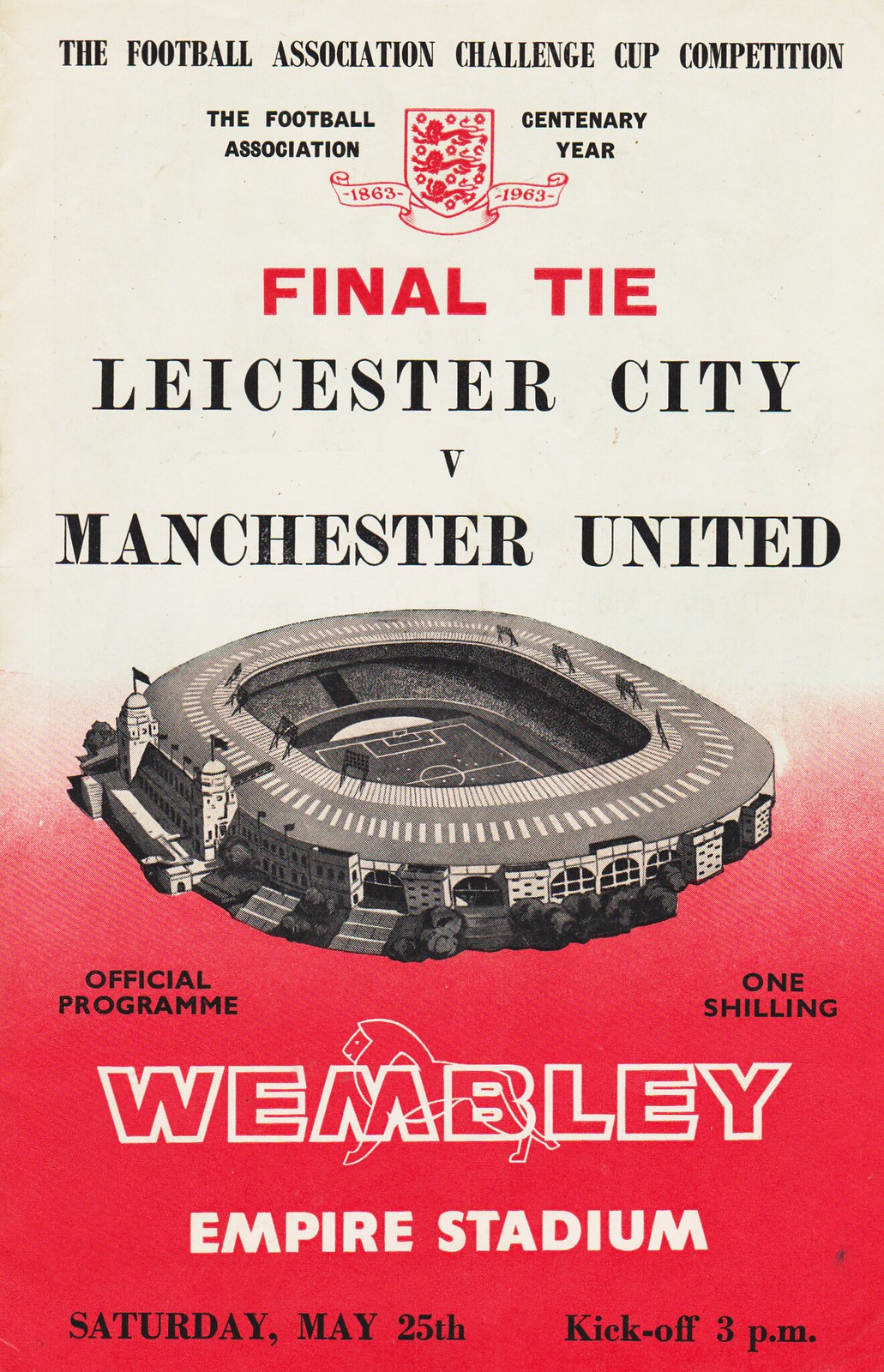This is a detailed poster for the Football Association Challenge Cup Accommodation, prominently displaying a striking white-to-red ombre background. At the top of the poster, the text reads "The Football Association Challenge Cup Accommodation." Below this, there is a distinguished Football Association emblem featuring a central shield flanked by two flags—one marked "1863" and the other "1963," signifying the centenary year. The text above this emblem states "The Football Association," while the right side displays "Centenary Year."

Beneath the emblem, the poster announces the "Final Tie: Leicester City v Manchester United." An illustration of a stadium, indicative of a soccer stadium, is prominently featured below this text. Further down, the poster identifies the venue as "Wembley Empire Stadium" and details the event specifics: "Saturday, May 25th, kick-off 3 p.m." 

Additional information includes that this is the "Official Program" priced at "One Shilling." The text is primarily in black, with select words highlighted in red and white, enhancing the visual emphasis and importance of key details.